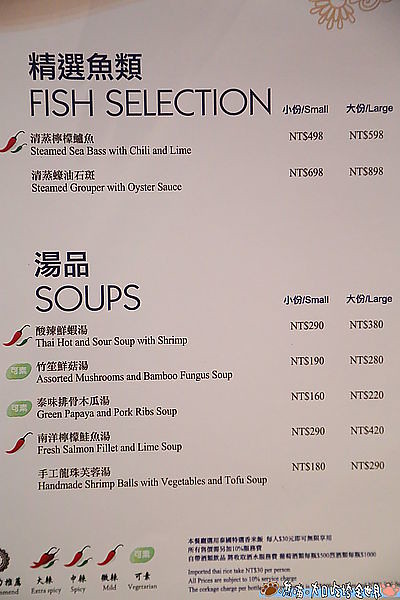The image depicts a menu, likely from an Oriental restaurant, featuring both English and Asian characters, potentially Japanese or Chinese. The menu is on an off-white background with sparse design elements. At the top, under Japanese characters, is the section titled "Fish Selection," listing items such as "Steamed Sea Bass with Chili and Lime" and "Steamed Grouper with Oyster Sauce." Prices for these items are shown in two columns for small and large portions, respectively, with options like NTS$4.98, $5.98, $6.98, and $8.98. Below this is the "Soups" section, which lists entries like "Thai Hot and Sour Soup with Shrimp," "Assorted Mushrooms and Bamboo Fungus Soup," "Green Papaya and Pork Rib Soup," "Fresh Salmon Filet and Lime Soup," and "Handmade Shrimp Balls with Vegetable and Tofu Soup," again indicating prices for small and large portions. The bottom part of the menu includes a legend detailing symbols for spice levels and dietary preferences, such as a chili pepper for mild and a green mark for vegetarian options. Additionally, there is some legal jargon and other information in Japanese located in the lower right corner.